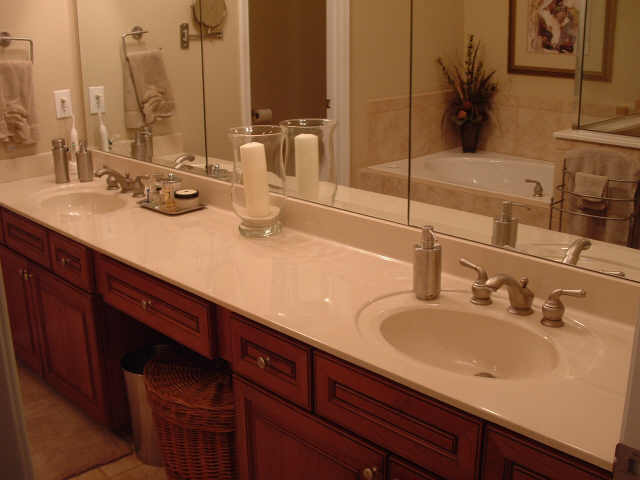This horizontal, rectangular photograph captures a meticulously styled bathroom interior, likely in a residential home. On the left side of the image, a section of a beige wall is visible, while the right side features a mirror affixed to the wall, reflecting additional elements of the room. Central to the composition is a long, elegant beige countertop that extends nearly the entire width of the image. Positioned symmetrically on the countertop are two sink bowls, each paired with stainless steel faucets and dual-handled fixtures.

Beneath the sinks, the cabinetry showcases rich, brown hardwood base cabinets, with each sink area featuring a double-door storage space. Additionally, there are five or six pull-out drawers aligned under the countertop, providing ample storage.

The mirror's reflection reveals more of the bathroom's layout, highlighting a white bathtub situated in the corner of the room. The bathtub is framed by beige wall tiles and accompanied by a lush green plant that adds a touch of nature to the space. Above the tub hangs an artwork in a brown frame, bordered with white edges and adorned with a floral design, contributing to the room's sophisticated decor.